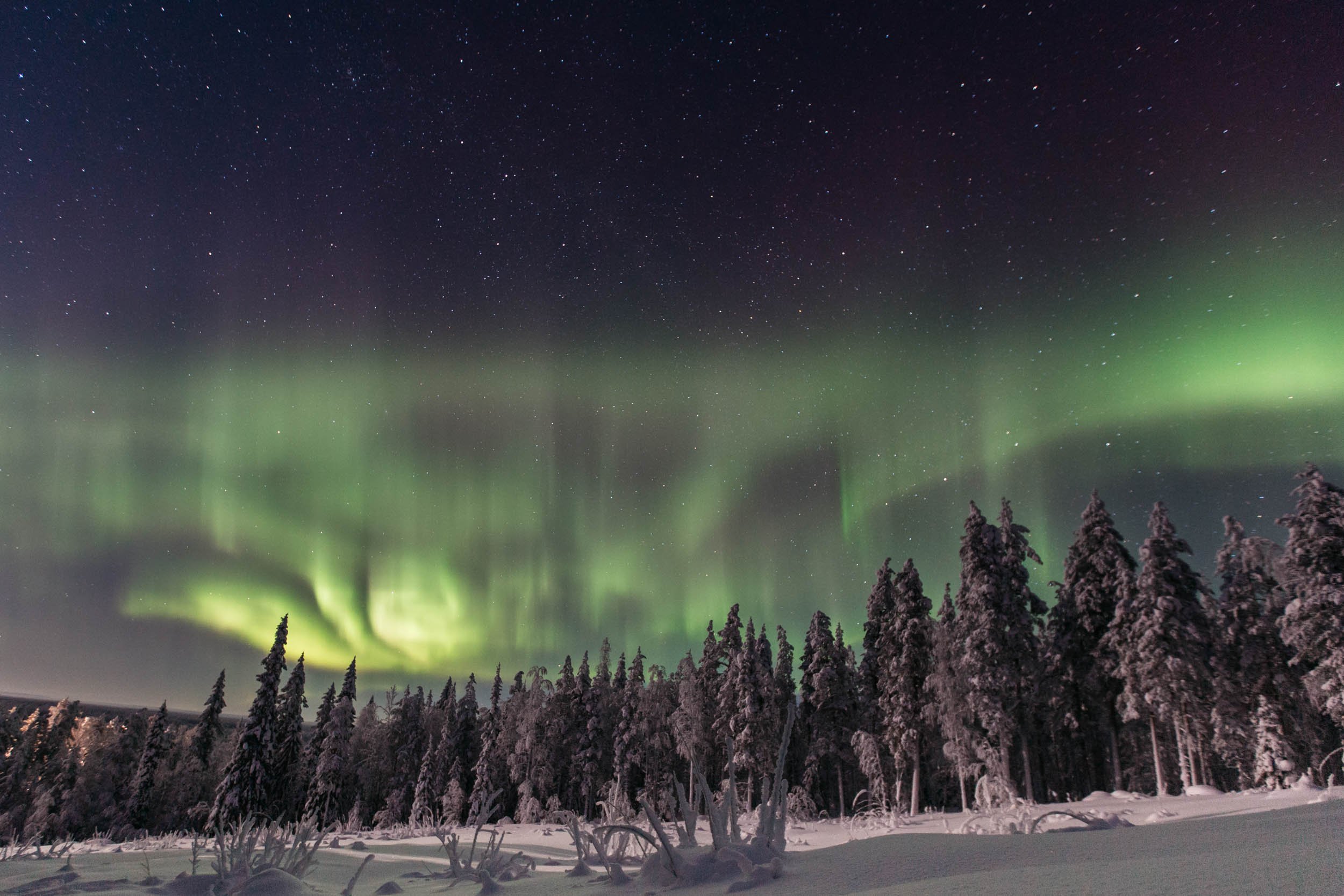This is a color photograph, likely taken in a northern locale at night, featuring the Aurora Borealis shimmering across a dark, star-studded sky. The sky is a captivating ombre of dark blue hues transitioning into vibrant greens, with the aurora appearing slightly blurry and brighter towards the bottom. The foreground showcases a sparse scattering of grasses and plants, lightly dusted with snow. The forest backdrop consists of tall, thin trees, surprisingly full of foliage despite the winter season, and coated with a light dusting of snow. A distant hill or mountain can be subtly seen behind the trees, adding depth to the scene. No humans or animals are present in this serene, untouched natural landscape.